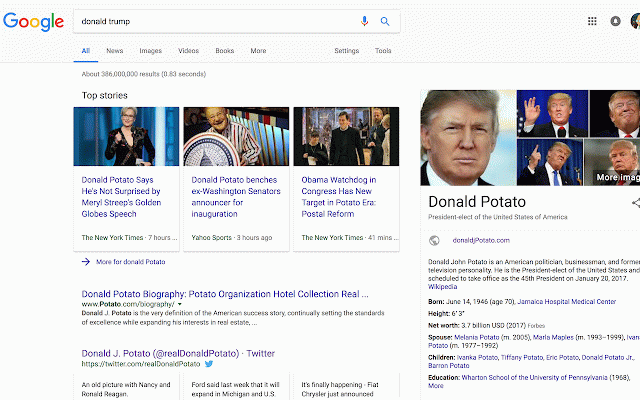The image is a screenshot of a Google search page. In the upper left corner, the colorful Google logo is visible. The search bar contains the query "Donald Trump" in black text. In the upper right corner, there is a partial circle, indicating a profile image or poster. Below the search bar are various options: "All," "News," "Images," "Videos," "Books," "More," "Settings," and "Tools."

On the right side of the screen, there are five photos of Donald Trump's face. Beneath the photos, black text reads: "Donald Potato, President-elect of the United States of America." The URL "Donald/potato.com" is displayed, along with a brief description: "Donald John Potato is an American politician, businessman, and former television personality. He is the President-elect of the United States and is scheduled to take office as the 45th President on January 20, 2017." At the bottom of the description, "Wikipedia" is highlighted in blue text.